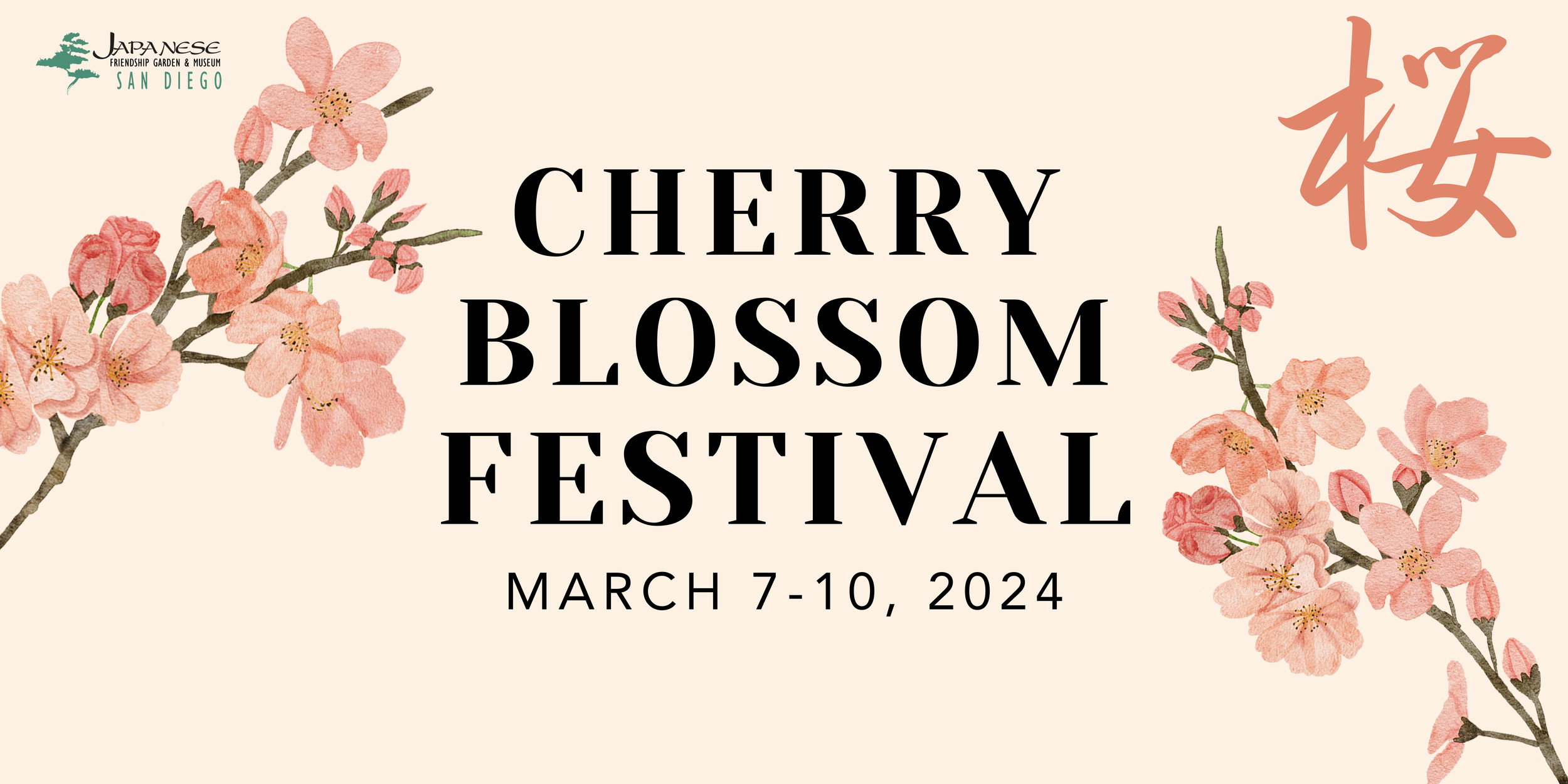This poster for the Cherry Blossom Festival, held from March 7 to 10, 2024, is predominantly designed in pastel and peachy-pink hues with floral elements that convey a serene atmosphere. Centered prominently in bold black font, the title "Cherry Blossom Festival" and the event dates stand out against a minimalistic beige background. The poster features two branches adorned with cherry blossoms, depicted in shades of pink and peach. These branches, complete with buds, add a realistic watercolor effect and traverse diagonally from the left and right sides of the title. In the upper right-hand corner, Japanese characters representing "cherry blossom" are inscribed, adding an authentic touch. The logo of the Japanese Friendship Garden and Museum in San Diego, resembling a bonsai tree, is positioned in the lower-left corner. The overall design emphasizes the floral theme with a balance of soft colors, incorporating both pink and subtle greenery.